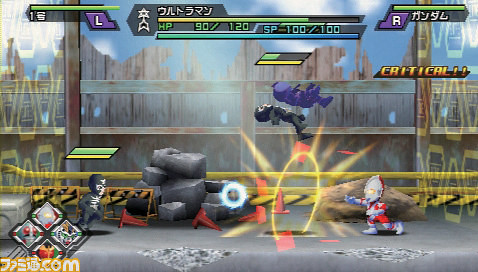The image is a detailed screenshot of a Japanese fighting video game. In the bottom left corner, there's a logo featuring the website URL "digio.com" in white lettering with orange highlights, positioned next to a diamond-like shape containing the faces of four robotic superhero characters. Prominent on the left side of the screen is a character wearing an all-black bodysuit with skeletal designs on the head and chest area. This character has a fully green health bar above a fully yellow secondary bar. To the right is a character in a red bodysuit with white markings who appears to be launching a fireball at the black-clad character. 

In the midst of the action, a large gray creature, reminiscent of a hippopotamus, looks to be in a punching pose with two characters and several orange street cones flying through the air, indicating a recent impactful attack. The word "critical" is displayed on the screen, suggesting a high-damage move. 

The scene includes a blue sky background with a partially destroyed large wooden fence, set above what appears to be a street-like ground. Additional details show green meters labeled "L" on the left and "R" on the right at the top of the screen. Various smaller graphical elements, like a circle with fire-like lights, enhance the portrayal of a dynamic and intense battle environment.